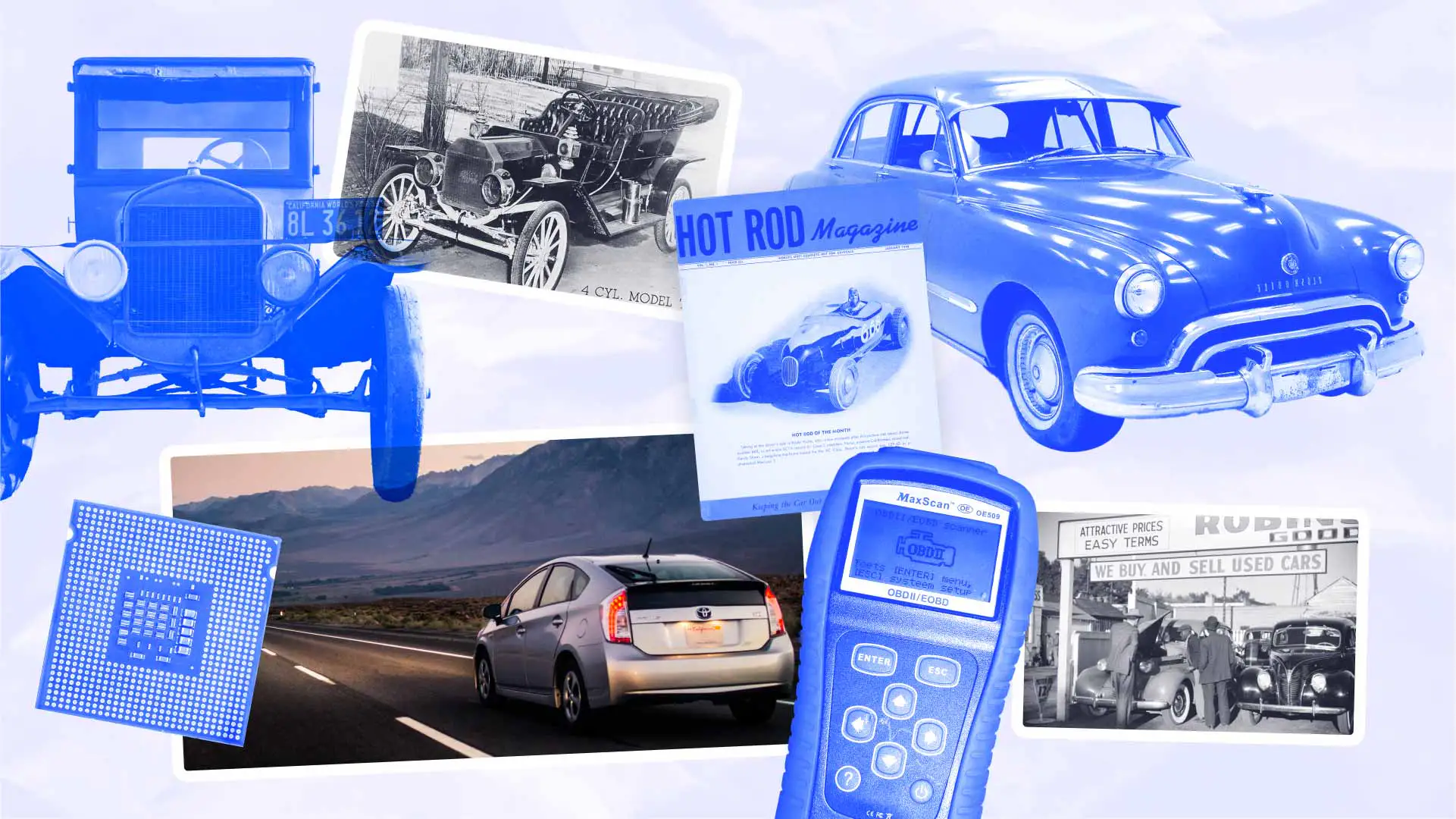This collage serves as a visual journey through the evolution of automobiles, spanning from early 20th-century models to modern vehicles. Set against a cloudy, light blue and white backdrop, the collage features a monochromatic blue arrangement of various eras in automotive history. In the upper left corner, there’s a blue-tinted image of a Model T or Model A, iconic for its vintage charm and narrow wheels. Just to its right, there is a grayscale photograph depicting another early 1900s automobile, possibly a Packard.

In the middle sits a vibrant blue cover of a "Hot Rod Magazine," showcasing a race car from the 1910s or 1920s, capturing the spirit of early automotive racing. Adjacent to this, a blue-hued rendition of a 1950s or 1960s family sedan, possibly a Studebaker, adds to the mid-century ambiance.

The lower portion of the collage highlights the transition to modernity. On the left, an actual silver Toyota Prius drives down a road, mountains framing the distant background, symbolizing the technological shift in automotive design. A small electronic device—likely an engine check tool—sits beneath this image, emphasizing the role of technology in modern vehicles. To its right, a microchip, also colored in blue, signifies the advancement of automotive engineering.

In the lower right, a black and white picture of a 1940s or 1950s car dealership provides a nostalgic glimpse into the commercial side of car history. Altogether, the collage not only showcases the aesthetic and technological progression of cars but also subtly references the tools and culture surrounding them.